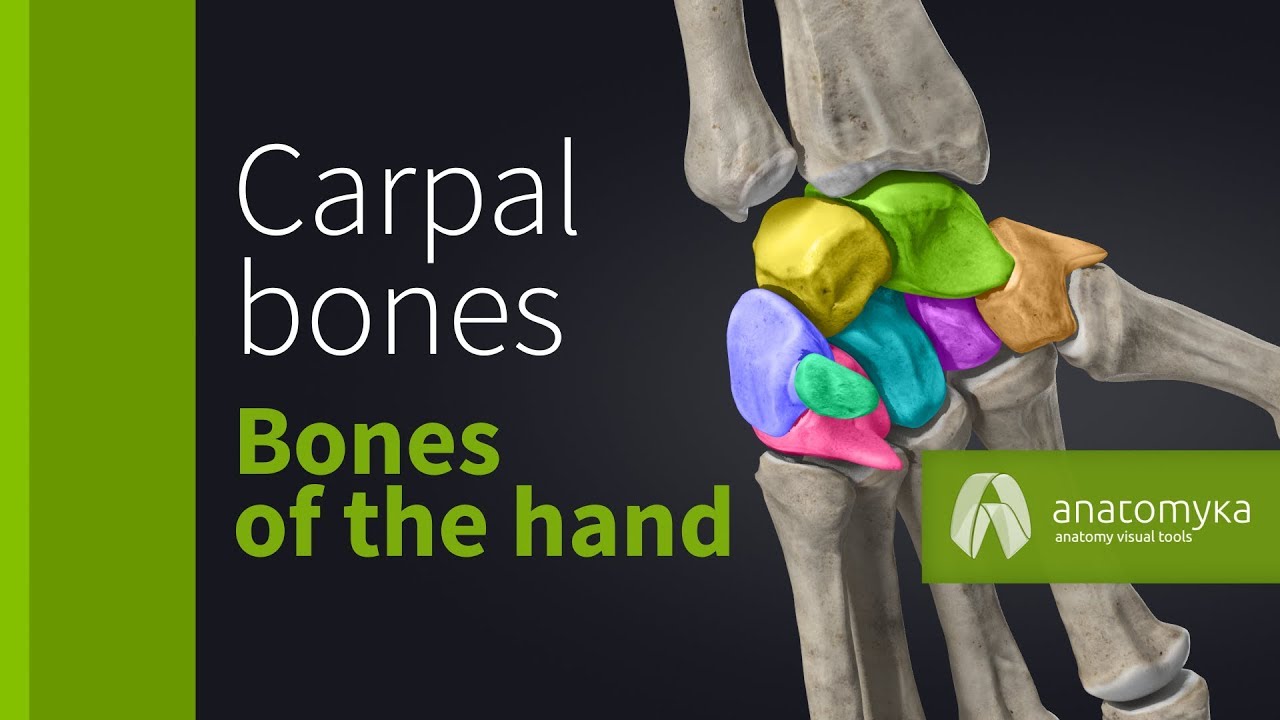The image depicts a color-coded, 3D skeletal representation of a human hand's bones against a black background with a gray gradient. On the left side, a green vertical stripe is bordered by a lighter green stripe, accompanying white text reading "carpal bones" and green text underneath stating "bones of the hand." Centrally and to the right, the hand bones are displayed with distinct colors: two upper bones, yellow on the left and green on the right; a second row from left to right, purple, green, pink, turquoise, dark purple, and light brown. A smaller green bone connects the purple and pink bones. Four elongated bones, representing fingers, extend downward from this central cluster. A green rectangle overlays the middle two finger bones. The right side includes a white stylized "A" logo, with the text "ANACOMYKA" and a tagline below reading "anatomy visual tools."